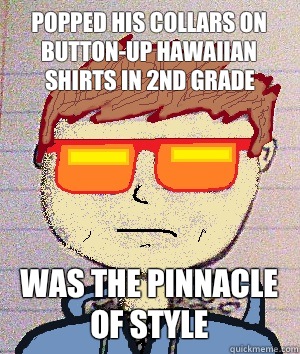The image depicts a large, bald, and bearded man with a muscular build, sitting or squatting on a bed covered with a red, gray, black, and white camouflage-patterned bedspread. He is wearing only a black jockstrap, with a visible tattoo on his right shoulder, possibly of a face. The man's expression is intense and somewhat smug as he looks up towards the viewer. His chest is hairy and his arms are positioned in front of him, partially obscuring his torso with a rolled-up black mat. The bed he sits on features black leather-like pillowcases and has a distinctive headboard behind him. The setting includes a window with gray blinds and gray walls flanking it. Central to the image, in bold, bright white text outlined in black, is the word "HAI," contributing to the photograph's unique blend of realism and representational typography.